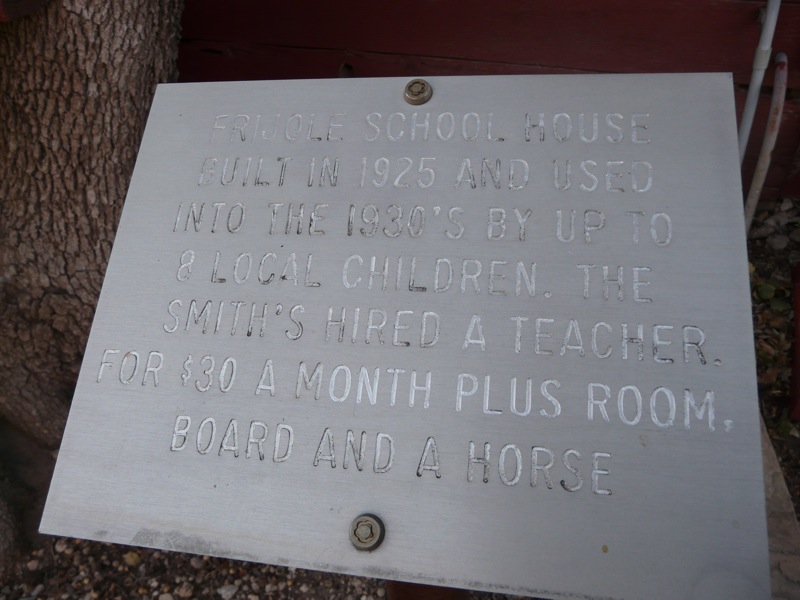This is a close-up image of an outdoor placard made of a worn, grayish silver metal that is engraved with historical information. The placard is secured with two large bolts, one at the top and one at the bottom, affixed either into the ground or onto a stand. The engraving on the placard reads: "Fresno School House, built in 1925 and used into the 1930s by up to 8 local children. The Smiths hired a teacher for $30 a month, plus room, board, and a horse." The surroundings include the partial image of a tree trunk to the left and some rocks on the ground beneath the placard, suggesting that it is in an outdoor setting. The background appears somewhat dark, possibly indicating it is located in front of a door or another structure, likely as part of an exhibit commemorating the old schoolhouse.